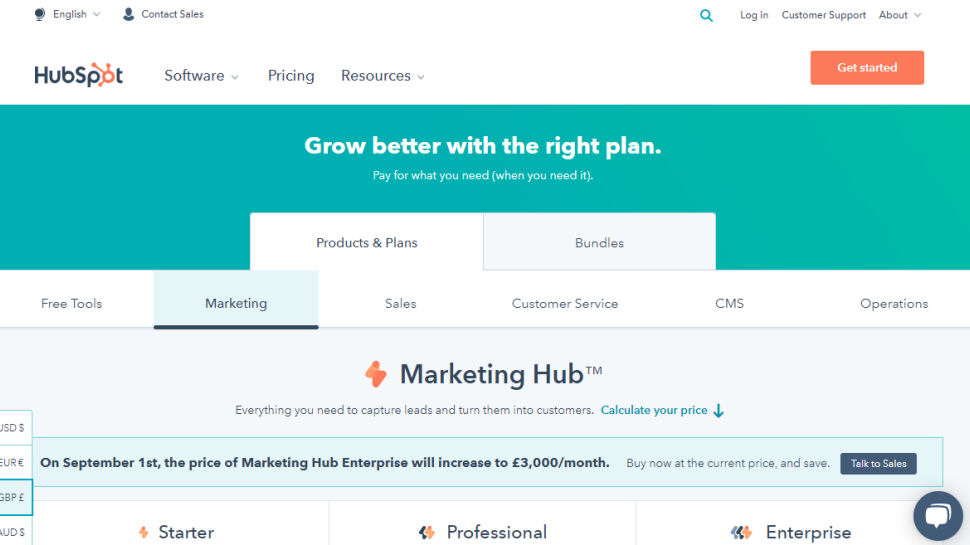**Detailed Caption:**

This image is a screenshot from the HubSpot website. The main HubSpot logo is prominently displayed at the top, with all its letters in black except for the letter "O," which is colored orange and adorned with several small lines ending in little balls, giving a distinctive design element. Adjacent to the logo, navigation options such as "Software," "Pricing," and "Resources" are listed in gray font. 

On the right side of the header, there is an English language icon with a drop-down menu, an option to "Contact Sales," and a placeholder image that likely represents a user profile which can be tagged. Additional options available in the header include "Customer Support" and "About," both with drop-down menus for further navigation.

Dominating the central area of the page is a box featuring a green-teal background. Inside this box, white text reads, "Grow better with the right plan. Pay for what you need when you need it." Beneath this, a header in white says "Products and Plans," and in gray text, it mentions "Bundles." 

The section below lists categories such as "Free Tools," "Marketing," "Sales," "Customer Service," "CMS," and "Operations," with the "Marketing" category highlighted. Upon highlighting "Marketing," the "Marketing Hub" details are revealed, stating, "Everything you need to capture leads and turn them into customers." 

A teal-linked drop-down menu provides the option to "Calculate your price." Below this, there is a time-sensitive notification indicating, "On September 1st, the pricing of Marketing Hub Enterprise will increase to €3,000 per month. Buy now at the current price and save." A prominent black button with white text prompts users to "Talk to Sales."

Lastly, the section lists tiers for various plans: "Starter," "Professional," and "Enterprise." At the bottom right corner, there is a chat box available for immediate customer assistance.